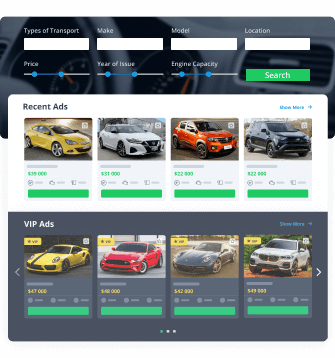A small square screenshot of a car buying website is displayed. At the top of the page, there are four white text fields labeled "Types of Transport," "Make," "Model," and "Location." Below these fields, interactive sliders allow users to adjust search parameters for "Price," "Year of Issue," and "Engine Capacity." A prominent green "Search" button is positioned beneath the sliders. 

The top section of the search area is overlaid onto a graphic resembling a gray dashboard. Directly below, a selection of vehicles is presented, divided into two categories. The "Recent Ads" section, featuring a white background, lists four cars with corresponding photos, each accompanied by a price and a button for additional information. Underneath, the "VIP Ads" section, set against a gray background, showcases four sports cars with similar details. The design is functional yet constrained by its small visual format.